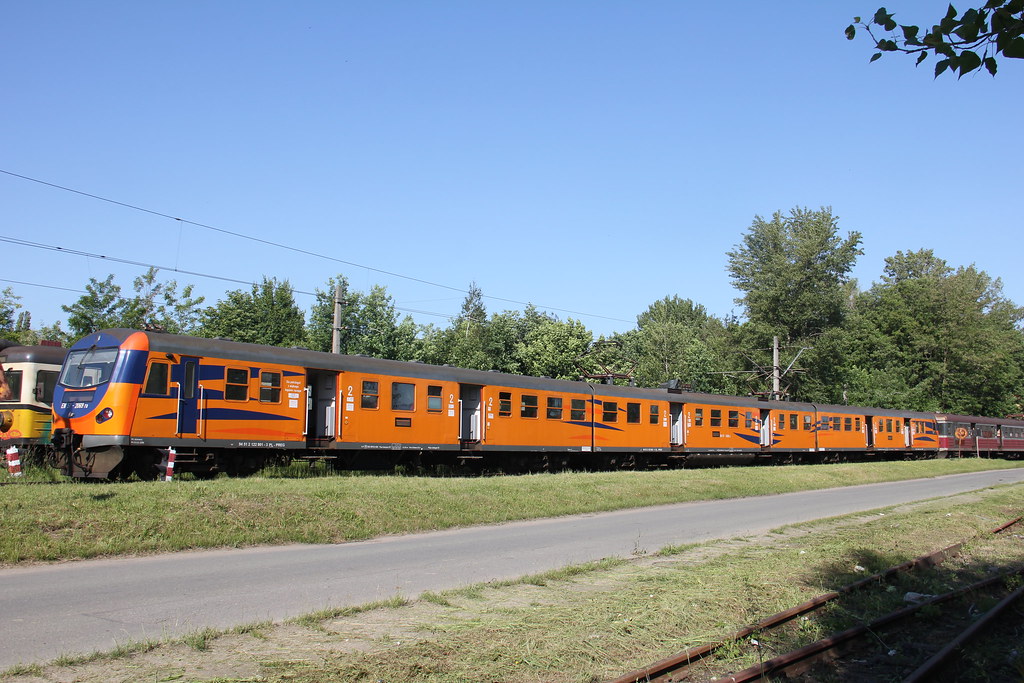The image captures a vibrant outdoor scene on a clear, sunny, blue-sky day without any clouds and only a few trees and power lines visible. Dominating the photograph, prominently positioned are modern, stationary trains. In the foreground, to the right, lie railroad tracks running parallel to a paved roadway. The first train, predominantly orange with a blue front and blue stripes, is coupled with multiple cars, of which at least eight are visible. It features handrails, steps, and three windows. In the distance, partially obscured, is a second train with its front in yellow and white. This train adds contrast to the scene, enhancing the dynamic feel of modern transportation infrastructure. The scene is completed with a roadside stand bearing a yellow circle and some tree limbs creeping into the right-hand corner of the frame.